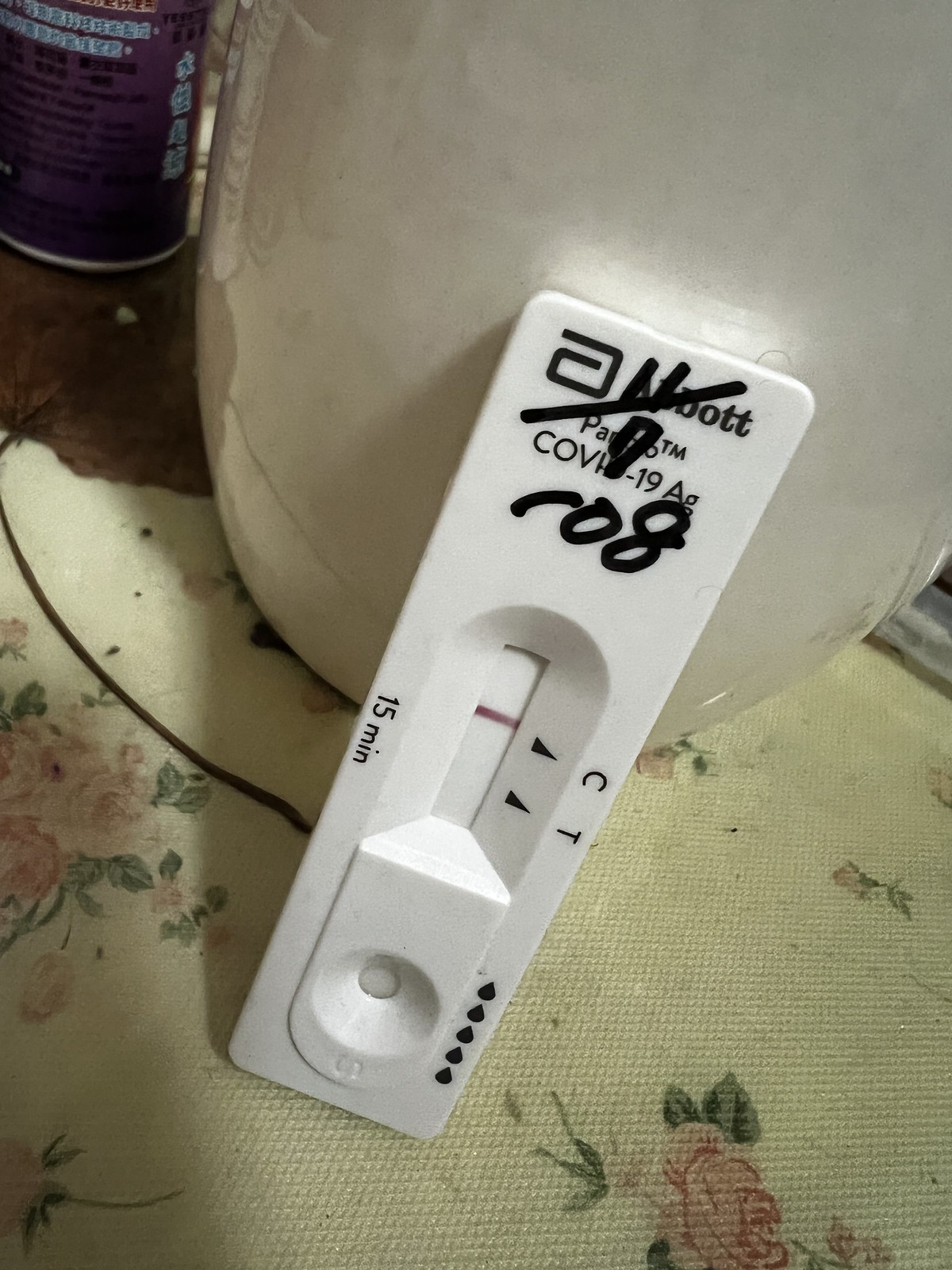The image features a COVID-19 test kit leaning against a vase on a table, which appears to be cluttered and dirty. The table is covered with a fabric or plastic material that has a rose pattern. The COVID-19 test kit, labeled "Abbott™ COVID-19 AG," has "N/7R08" written over it in black Sharpie. In the background, there is a purple can and a brown leaf, positioned so that the stem of the leaf points back towards the test kit. The test kit reveals a single red line at the "C" marker, indicating a negative result, provided that the full 15 minutes have elapsed. The test instructions specifying "15 minutes" are also visible on the kit.